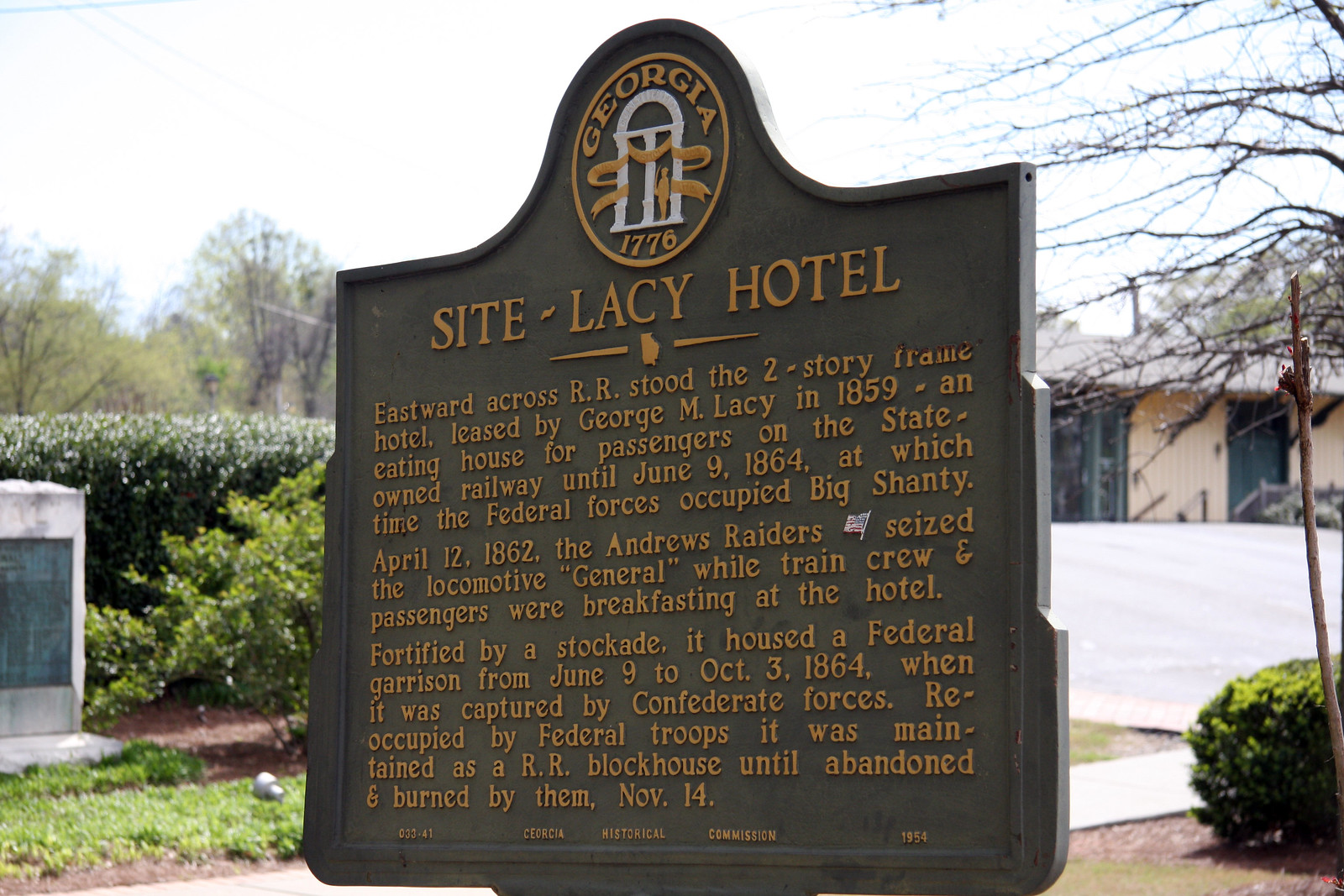The photograph features a prominent outdoor historical marker titled "Site Lacey Hotel," located in Georgia. The large, dark-colored sign, set against a backdrop of greenery, includes detailed golden text recounting the site's history. The Lacey Hotel, a two-story frame building leased by George M. Lacey in 1859, served as an eating house for passengers on the state-owned railway until June 9, 1864. During the American Civil War, it became notable for the Andrews Raiders' seizure of the locomotive General on April 12, 1862. The hotel, later fortified and housing a Federal garrison, shifted hands multiple times until it was ultimately burned by Federal troops on November 14. Behind the sign, a bit of the hotel and a white fence or wall are visible, along with a well-kept border of green shrubbery, trees, and a sky that appears white. The detailed historical marker, complemented by its serene surroundings, stands as a testament to the rich past of the area.